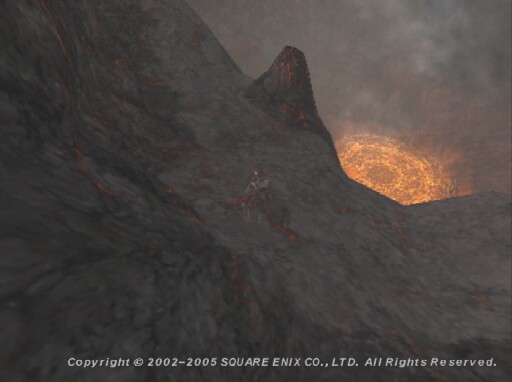This image is a blurry, colour screenshot from an older video game, possibly from the PlayStation 2 era, and it is not very appealing. The scene depicts a dark, rocky, and potentially volcanic mountain range, characterized by a palette of dark gray, black, brown, and hints of red. At the bottom of the image, in white text, it reads "Copyright 2002-2012 Square Enix Co. Ltd. All rights reserved." A major focus of the image is a very large, fiery, oval sun either setting or rising over the mountain peaks, casting an indistinct light that creates the illusion of spokes emanating from it. The sky is dominated by dark gray clouds, adding to the bleak atmosphere. Within this setting, there appears to be a barely visible human-shaped figure, possibly clad in gray and red armor with a backpack. The overall scene conveys a sense of desolation, with the mountain descending into what looks like a pit of lava or a volcano, further emphasizing the harsh, unwelcoming environment.